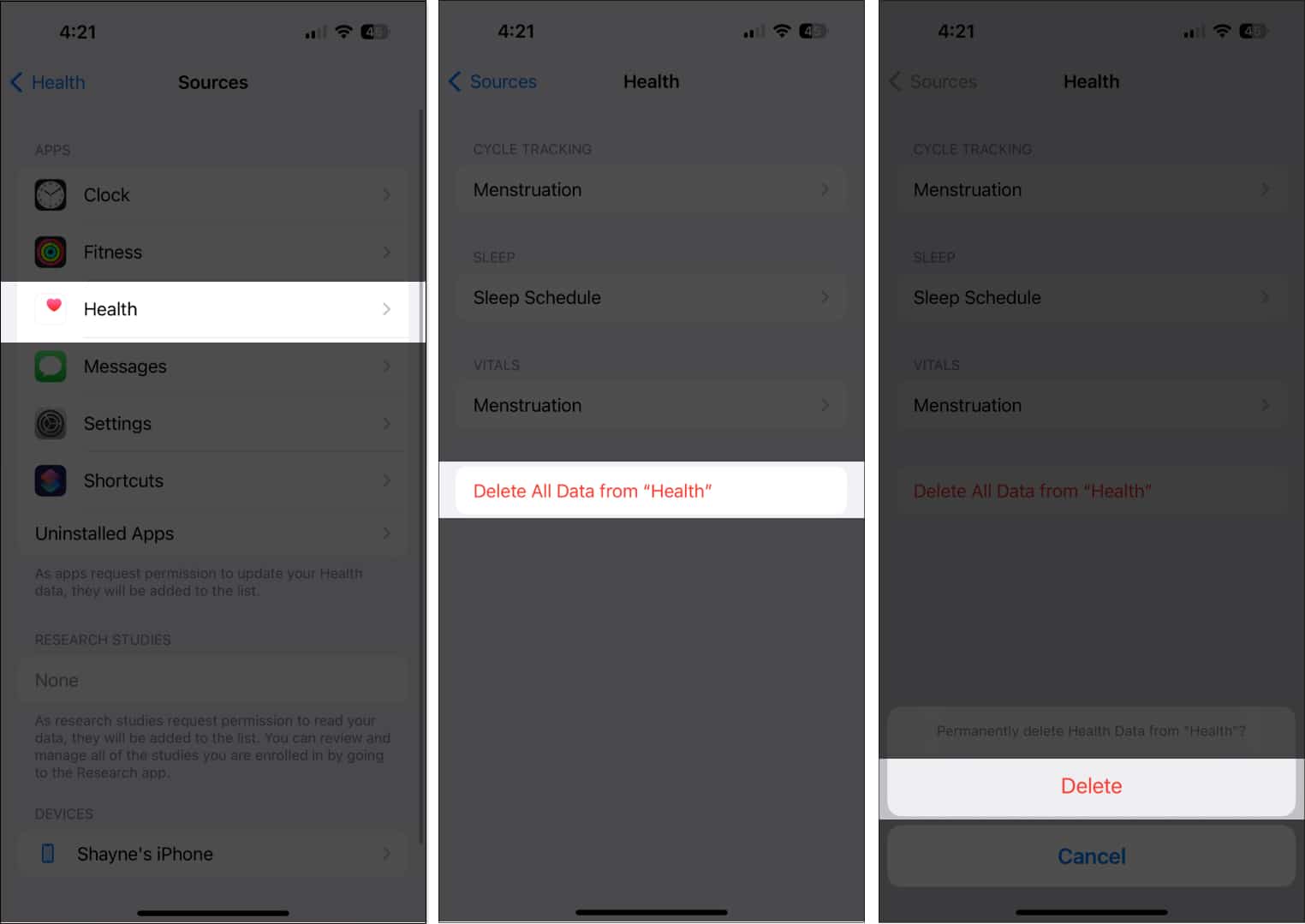**Detailed Caption**

This triptych of mobile application screenshots illustrates the process of navigating to and deleting health data. Each screenshot features a primarily darkened page with a highlighted rectangular area that draws focus.

1. **Left Screenshot**: The highlighted area, positioned near the top, reveals a white rectangle with a light gray right-pointing arrow on its right side. To the left of the arrow is a pink heart icon, accompanied by the word "Health" in black text. The title centered at the top reads "Sources" in bold black text, with "Health" and a left-pointing blue arrow situated in the top left. The timestamp in the top left corner is "4:21". The background has a slightly purplish tint.

2. **Middle Screenshot**: Here, the highlight is located halfway down the page, illuminating another white rectangle. Inside, red text states, "Delete all data from 'Health'". The title at the top center reads "Health" in bold black text. To the left of the title is the word "Sources" with a left-pointing blue arrow. Like the previous screenshot, the time displayed in the top left corner is "4:21". The overall background remains purplish.

3. **Right Screenshot**: In this image, the highlight is near the bottom fifth of the page, showcasing a white rectangle with rounded bottom corners containing red text that reads "Delete". The top center title still reads "Health" in bold black text. Unlike the previous screenshots, the top left displays the word "Sources" with a gray arrow, both in gray text. The timestamp remains consistent at "4:21". The background continues with a purplish hue.

Across all screenshots, additional white rectangles containing various texts are visible, reinforcing uniformity with a purplish-tinged dark background.